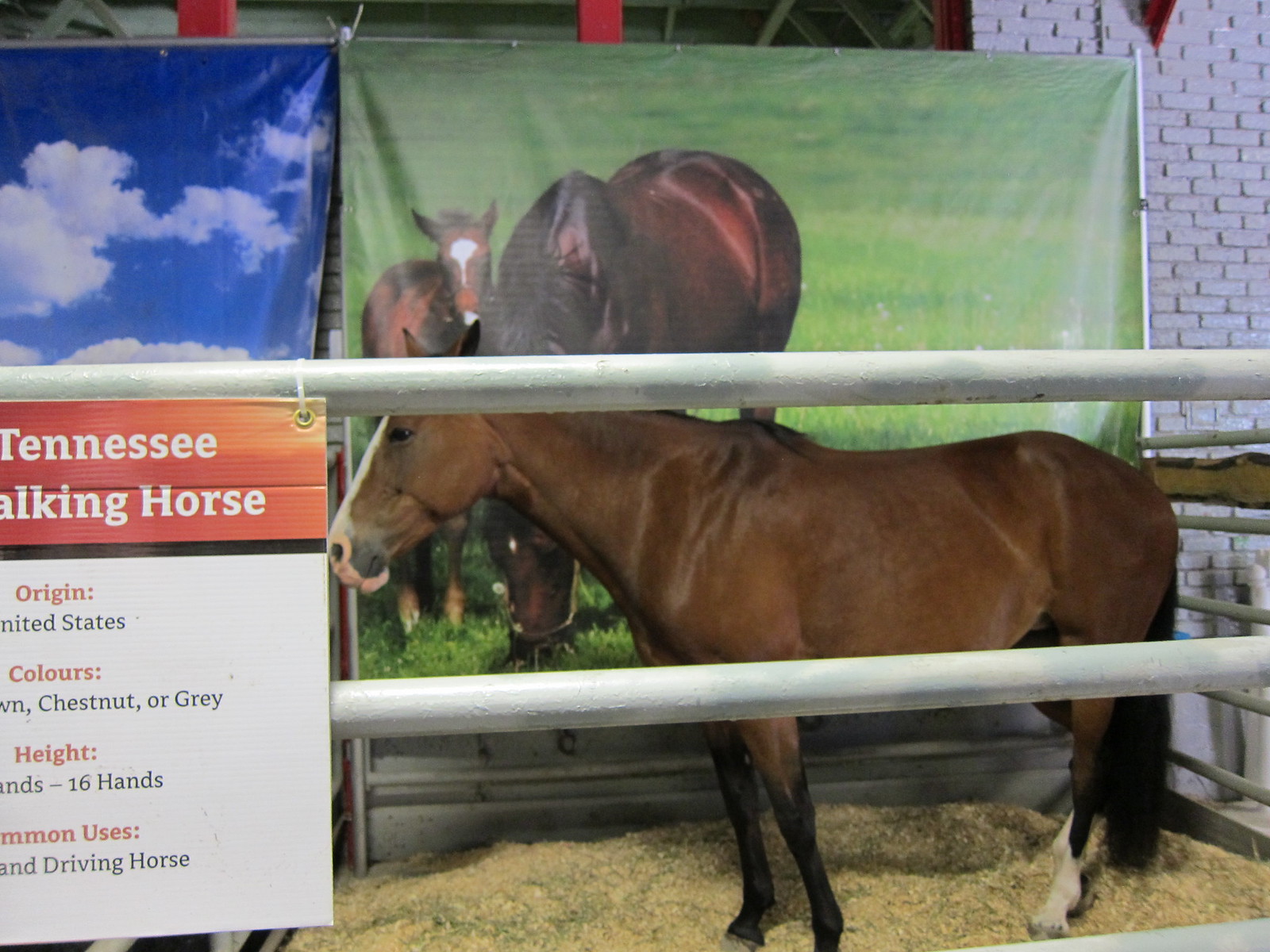The image features a brown Tennessee Walking Horse standing sideways in a metal stable. The horse has a distinctive white stripe down its forehead and a pinkish nose, with blackish legs, tail, and mane. It is standing on a flooring covered in hay. In the foreground, there is a detailed sign zip-tied to the stable railing. The sign has a red stripe at the top, followed by black and white sections. Although partially obscured, the sign provides information such as the horse's origin (United States), available colors (brown, chestnut, and gray), height (16 hands), and common uses including driving. Behind the horse, there are tarpaulin posters, one depicting a mother and baby horse grazing in a field with a blue sky and white clouds, and the other showing a serene grass field. The stable itself is enclosed by steel bars, with a backdrop of gray brick walls. The horse appears to be looking down, creating a somewhat somber ambiance.